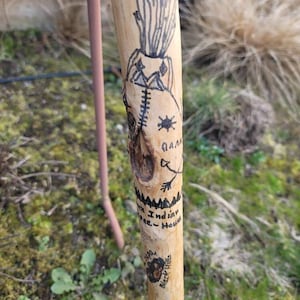The photograph captures a small wooden pole or stick, likely a smooth tree branch, embedded in the ground amidst a mix of grass, weeds, and dry bushes. The light yellowish-blonde wood features simple, black marker drawings and patterns, possibly resembling native artwork or graffiti done by children. The legible portion includes the word "Indian" among other symbols and potentially figures. The background is blurred, but showcases a variety of greenery in shades of light, dark, and regular green, interspersed with dry, light brown vegetation, suggesting the photo was taken outdoors during the day.